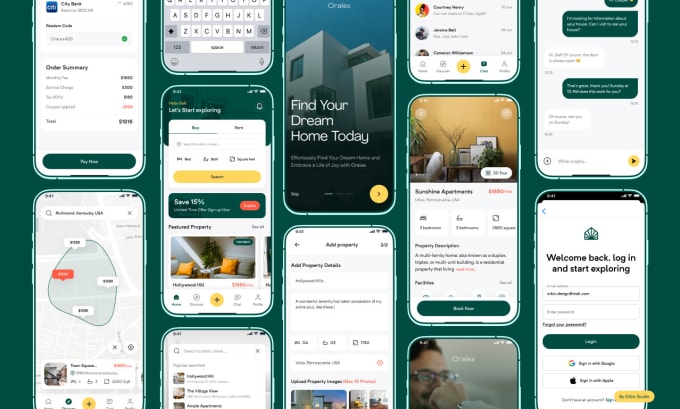A visually striking promotional image for a real estate app, prominently features a smartphone in the center. The top-left corner showcases a vibrant blue element, contrasting with white spaces and bold red accents. In December, a significant textual area replaces paint, enhancing readability and impact. Below, there are multiple smartphones depicted, highlighting user-friendly interfaces. A virtual keyboard suggests interactive features for property searches.

In the middle of the image, a large green area with rounded edges provides a calm background. The top of this section contains the encouraging text "Find your dream home today" in bold. A conspicuous yellow circle with the prompt "Add Property" catches the eye. Additional text and images are scattered throughout, with white backgrounds making the information stand out.

At the bottom of the image, more green areas seamlessly blend with white sections, enclosing photos and text. One picture shows a pair of glasses, perhaps hinting at detailed viewing options available within the app. Black and white bars at the edges frame the image, giving it a modern, sleek look.